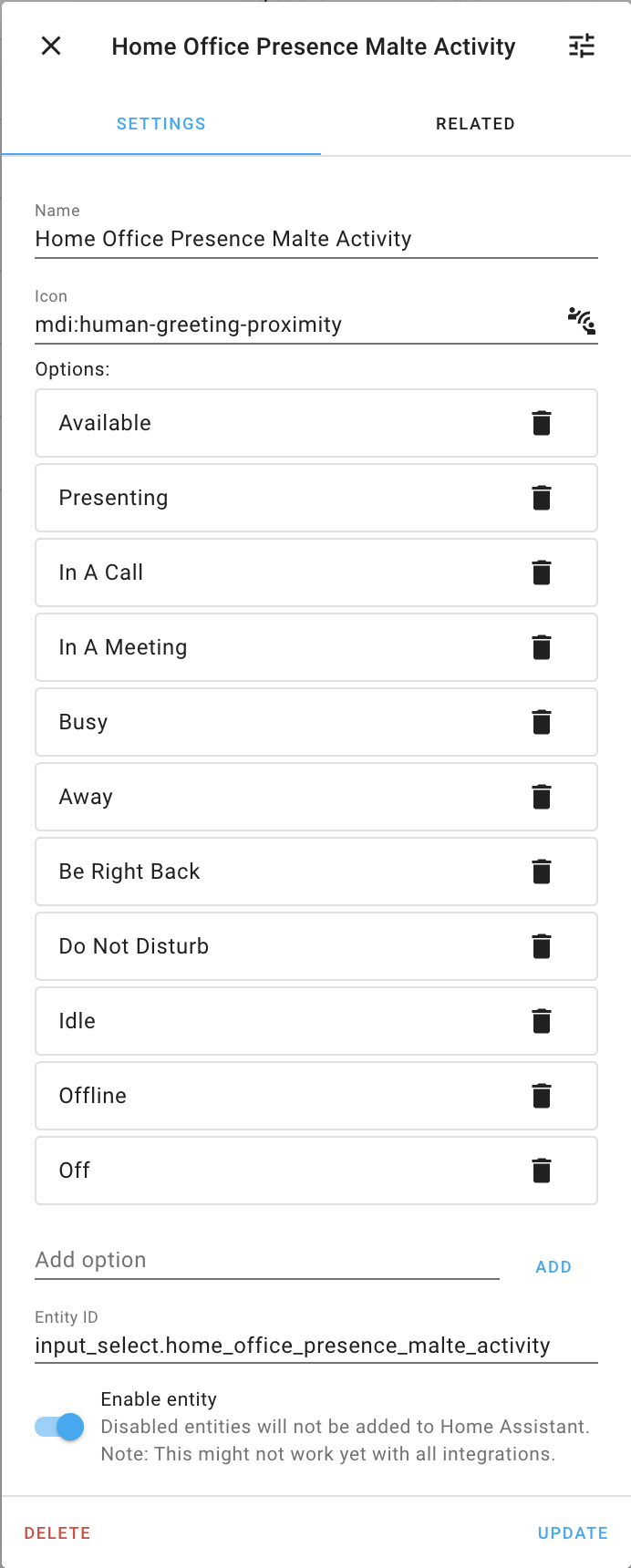This image appears to be a section from a larger interface printout related to managing presence in a home office setting. The heading at the top reads "Home Office Presence Multi-Activity." Directly below, the same heading is repeated. 

Under the main heading, there’s a segment labeled "ICON" with the descriptor "MDI: human-greeting-proximity," followed by an unspecified symbol. The page lists various status options, each accompanied by a trash bin icon for discarding. The available statuses include:

- Available
- Presenting
- In a Call
- In a Meeting
- Busy
- Away
- Be Right Back
- Do Not Disturb
- Idle
- Offline

Additionally, there is an option to add a new status labeled as "empty ID input_select.home-office-presence-multi-activity." At the bottom, there’s a toggle for an "Enable Entity" button, which appears to be switched on.